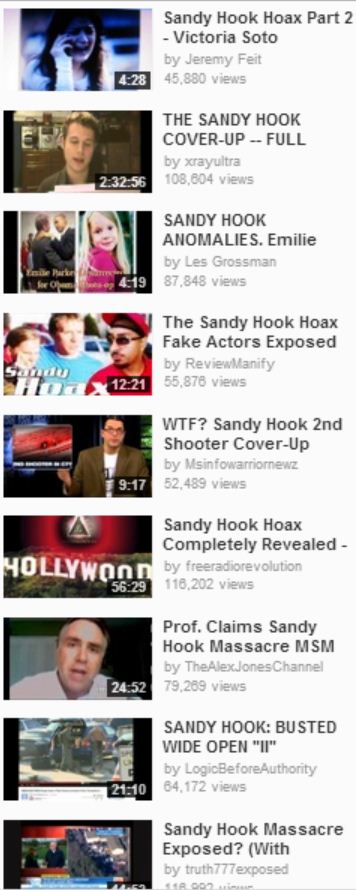The screenshot, taken from a vertically long mobile device, displays a collection of nine videos related to Sandy Hook. Each video is presented with a title, thumbnail, uploader information, view count, and duration. 

1. **Sandy Hook Hoax Part 2 Victoria Soto** by Jeremy Fate – 45,880 views, 4 minutes 28 seconds.
2. **Sandy Hook Cover-Up – Full** by x-ray ultra – 108,604 views, 2 hours 32 minutes 56 seconds. The thumbnail features a white man with a brown background, reading from a piece of paper.
3. **Sandy Hook Anomalies: Emily** by Les Grossman – 87,848 views, 4 minutes 19 seconds. Les Grossman is noted as a famous author.
4. **WTF? Sandy Hook Second Shooter Cover-Up** by Miss Info Warrior News – 52,489 views, 9 minutes 17 seconds.
5. Another four videos focused on various aspects of Sandy Hook, including theories of hoaxes and analyses by professors, rounding out the collection.